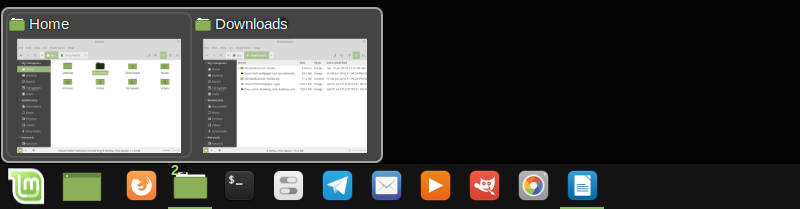The image depicts a computer desktop with a black background. On the left side, there are two prominent folder pop-ups. The top folder is labeled "Home" with a green folder icon and the contents of the folder include several individual items, though the specific details are too small to read. Below it is another folder labeled "Downloads", similarly marked with a green folder icon, showing items populated within it. Both folders have a black legend with white writing that is difficult to decipher due to its size.

At the bottom of the screen, there is a series of 12 icons representing different applications and functions. From left to right, they include a green icon with letters that resemble "LM", a green rectangle, an orange icon possibly representing Firefox, a folder icon labeled with the number 2, a black icon featuring a dollar sign, a white icon symbolizing switches against a blue background, a blue icon with a white paper airplane design possibly indicating Telegram, a blue icon with a white envelope denoting email, an orange icon with a white play triangle, a red icon with a stylized face, a gray icon representing a camera lens, and a blue icon with a graphic of a paper containing writing. The overall interface suggests an active and organized digital workspace.